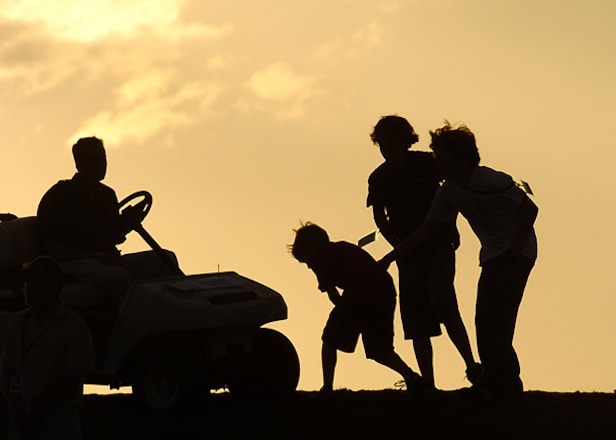The photo is taken outdoors at sunset, featuring the silhouetted figures of three boys and a man seated on a small four-wheeled vehicle, possibly a golf cart or lawnmower. The smallest boy is hunched over, wearing shorts and a short-sleeved shirt, while the other two taller figures stand close by, almost appearing to have their arms around the youngest. All the figures are in complete black silhouette against a hazy beige-gray sky, illuminated by the golden glow of the sun, lending a surreal quality to the scene. The exact activity captured in the image is ambiguous, but the tableau suggests a moment of play or companionship.